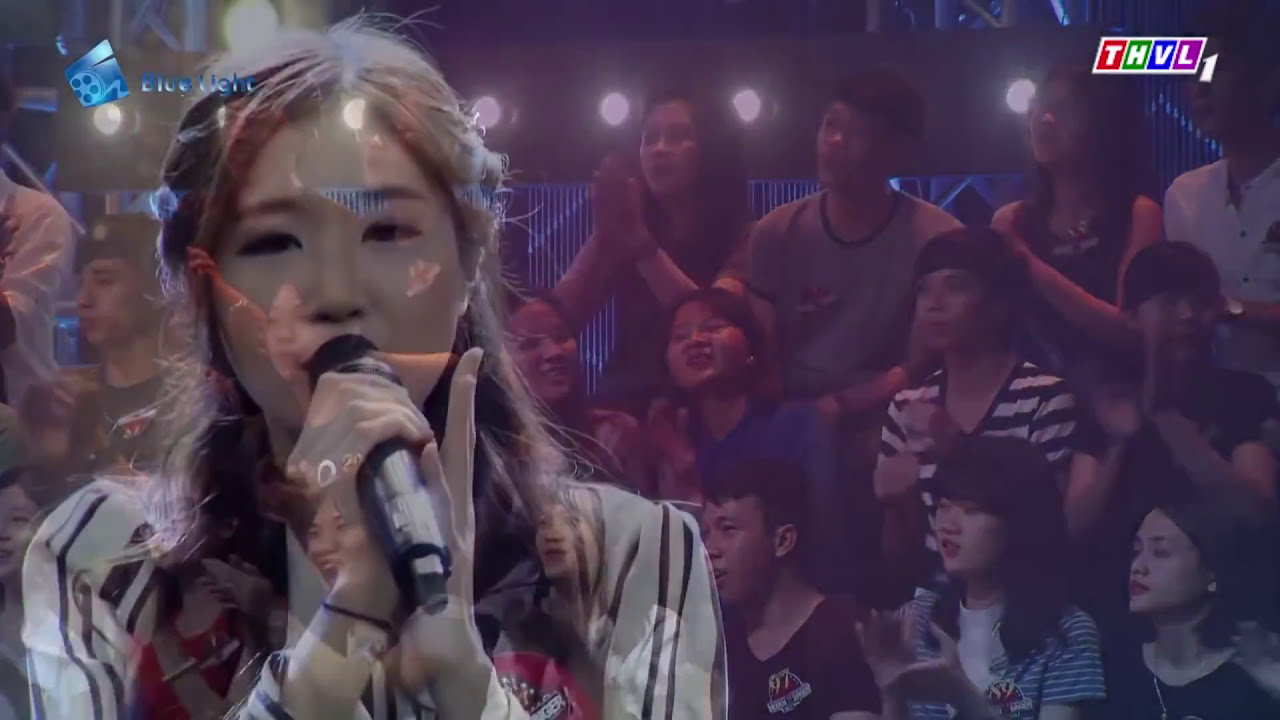The image is a detailed screenshot from a TV show or contest, featuring a blend of two scenes. The background shows a large, enthusiastic audience of primarily Asian individuals, seated in three rows within a room bathed in purple and blue lighting. They appear captivated, all clapping and looking towards the left side of the image. Overlaid on this background is a transparent, prominent image of a young Asian woman singing into a microphone. She has shoulder-length, somewhat curly blond hair, and distinctive pale skin. She wears a red shirt with black and white striped sleeves, and her dark-colored eyes are open as she performs. In the upper right corner of the image, there's a graphic with the letters "THVL" in white, placed within red, green, blue, and purple boxes. Additionally, the upper left corner features the word "blue" written in blue text. The photograph captures a moment of shared enjoyment and focus, highlighting both the performer's intensity and the audience's engagement.